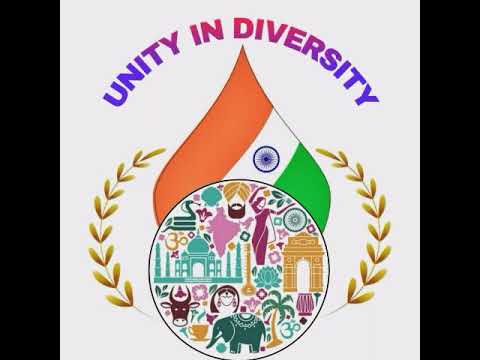This digital image features a central logo set against a white background, framed by solid black borders on both sides. At the top of the image, the text "Unity in Diversity" is prominently displayed in vibrant blue and red colors. Below this, the logo itself is centered, comprising two main elements: a circle filled with diverse, colorful illustrations and a teardrop-shaped motif behind it, representing the Indian flag with its orange, white, and green stripes.

Within the circle, there is a rich tapestry of detailed imagery symbolic of Indian culture, including a blue elephant, the face of a cow, and a man in a yellow headdress. Additionally, a woman in purple appears to be dancing akin to a Bollywood performer, and there are depictions of iconic Indian landmarks like the Taj Mahal in a light teal color. Also included within the circle are drawings of a palm tree, a purple map of India, and other intricate elements that collectively celebrate the theme of India's unity in diversity.

Surrounding the circle and the teardrop are elegantly designed golden leaves that spiral upwards, adding an ornate touch to the overall design. The composition of the image, with its melding of colorful and culturally significant visuals, appears to be intended as an inspirational message suitable for sharing on social media.